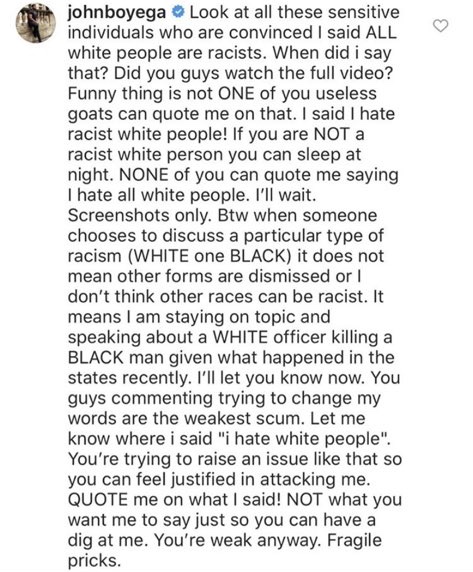**Image Description:**

A vertical image containing a block of text.

- On the left-hand side, there is a black and white image inside a circle, though the details are unclear.
- Adjacent to the circle, in bold black font, is the name "John Boyega."
- Next to his name, there is a turquoise circle with a white check mark inside.

**Text Details:**

The body of the text is in regular black font (not bolded):

"Look at all these sensitive individuals who are convinced I said ALL (capitalized A-L-L) white people are racist. When did I say that? Did you guys watch the full video? Funny thing is, not ONE (capitalized O-N-E) of you useless goats can quote me on that. I said, I hate racist white people. If you are NOT (capitalized N-O-T) a racist white person, you can sleep at night. NONE (capitalized N-O-N-E) of you can quote me saying, I hate all white people. I'll wait. Screenshots only. BTW, when someone chooses to discuss a particular type of racism (WHITE, BLACK), it does not mean other forms are dismissed or that I don't think other races can be racist. It means I am staying on topic and speaking about a WHITE officer killing a BLACK man, given what happened in the States recently. I'll let you know now, you guys commenting and trying to change my words are the weakest scum. Let me know where I said, 'I hate white people.' You're trying to raise an issue like that so you can feel justified in attacking me on what I said, NOT (capitalized N-O-T) what you want me to say, just so you can have a dig at me. You're weak anyway, fragile, and then an inappropriate word. There is also an unfilled heart icon at the top of the post."

This highly detailed caption effectively conveys both the visual and textual elements of the image, providing a comprehensive description.